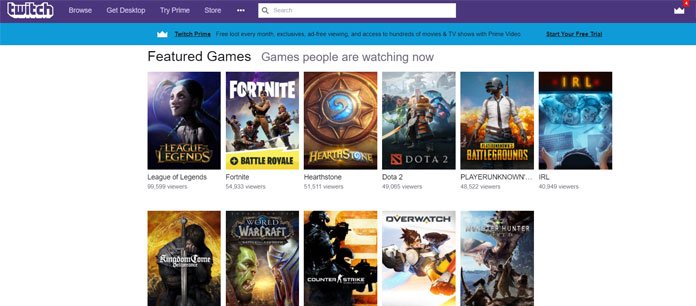This image features a webpage with a predominantly white background. At the top, there is a purple banner with the Twitch logo in white. The banner also includes the text "Browse," "Get Desktop," "Try Prime," and a set of three vertical white dots (likely a menu icon). 

To the right of this banner, there is a search bar, followed by a white crown icon with a small red notification box above it, containing a white number.

Below the banner, on the left side, there is a blue box featuring a white crown icon and the text "Twitch Prime." This section promotes a free trial for Twitch Prime, displaying options to "Start Your Free Trial."

The main content area of the page showcases various game titles under the headers "Featured Games" and "Games People Are Watching Now." The top row includes six game titles: "League of Legends," "Fortnite Battle Royale," "Hearthstone," "Dota 2," "PLAYERUNKNOWN'S Battlegrounds," and "IRL." 

Below this row, there are four additional games listed, including "World of Warcraft," "Overwatch," and a game with a partially legible title that seems to include the word "Hunter." One title in this row is too small to be read clearly. 

The overall layout of the image suggests that it is the landing page of a gaming and streaming platform, with a focus on popular games and promotional content for Twitch Prime.